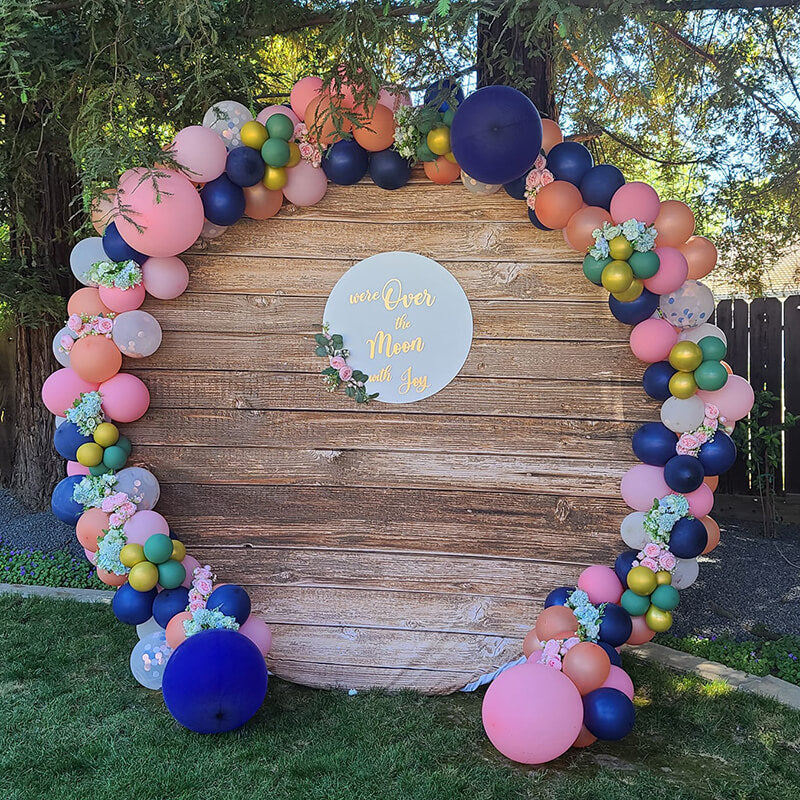The photograph depicts an outdoor backyard scene during the daytime, framed with green grass and bordered by wood edging and graystone gravel. To the left, a tall tree with a brown trunk and lush green leaves stands out, while to the right, there's a wooden fence with the blue sky visible through its gaps and tree branches. 

At the center of the image lies a circular structure crafted from horizontal wooden planks, resembling a tabletop, with an overall diameter of approximately six inches. Positioned in the middle of this wooden circle is a smaller, light gray-colored circle inscribed with golden cursive text reading, "we're over the moon with joy," with "over the moon" notably larger than the rest of the phrase. 

The lower left quadrant of the circle, roughly between the 6:30 and 9:00 positions, is adorned with green leaves and two small pink roses. Surrounding the wooden circle is a festive array of colorful balloons and flowers. The balloons come in shades of pink, blue, green, yellow, and some occasional orange, along with smaller elements like gold and even clear balloons. Scattered among the balloons are blue and pink flowers, including what appear to be carnations, creating a vibrant and celebratory display.